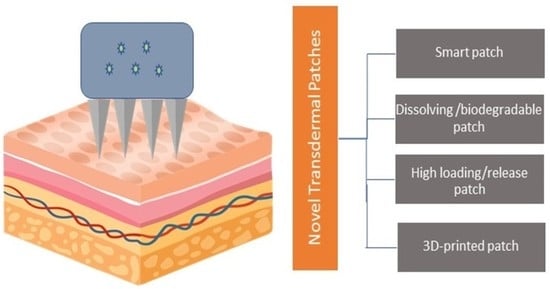This detailed illustration, likely found in a dermatologist's office, shows a diagram of novel transdermal patches against a white background. To the left is a detailed representation of human skin layers. The bottom layer features a mustard yellow tone with light tan blobs, above which lies a tan layer interwoven with wavy red and dark blue lines. Above that is a pinkish-tan layer, followed by a thin white layer, and then a slightly darker pink layer. The topmost layer is tan-colored, representing the epidermis. On this epidermal layer sits a gray rectangle with five star-shaped points and four triangular spikes projecting downwards.

To the right of this skin illustration is an orange rectangle labeled "novel transdermal patches," connected by lines to four gray boxes. These boxes are titled "Smart Patch," "Dissolving Biodegradable Patch," "High Loading Release Patch," and "3D Printed Patch." The entire setup seems to convey how these advanced patches interact with and penetrate the skin layers, highlighting their benefits and functionalities.